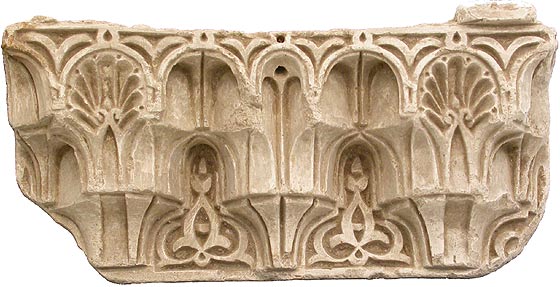This photograph showcases an intricately detailed architectural element, possibly made of stone, plaster, or limestone. The piece is a light beige or cream color with white highlights, depicting a delicate balance of depth through its carved patterns. The design features elegant curves, arches, and scrolls that reflect a historical or ecclesiastical influence, with hints of Celtic style in the swirled cutouts at the bottom. Two shell or peacock-like engravings and three cone-shaped motifs add to its ornate beauty. This rectangular, yet slightly chipped, piece exemplifies meticulous craftsmanship, bearing varied etching depths that highlight the complexity and artistic dedication involved in its creation.